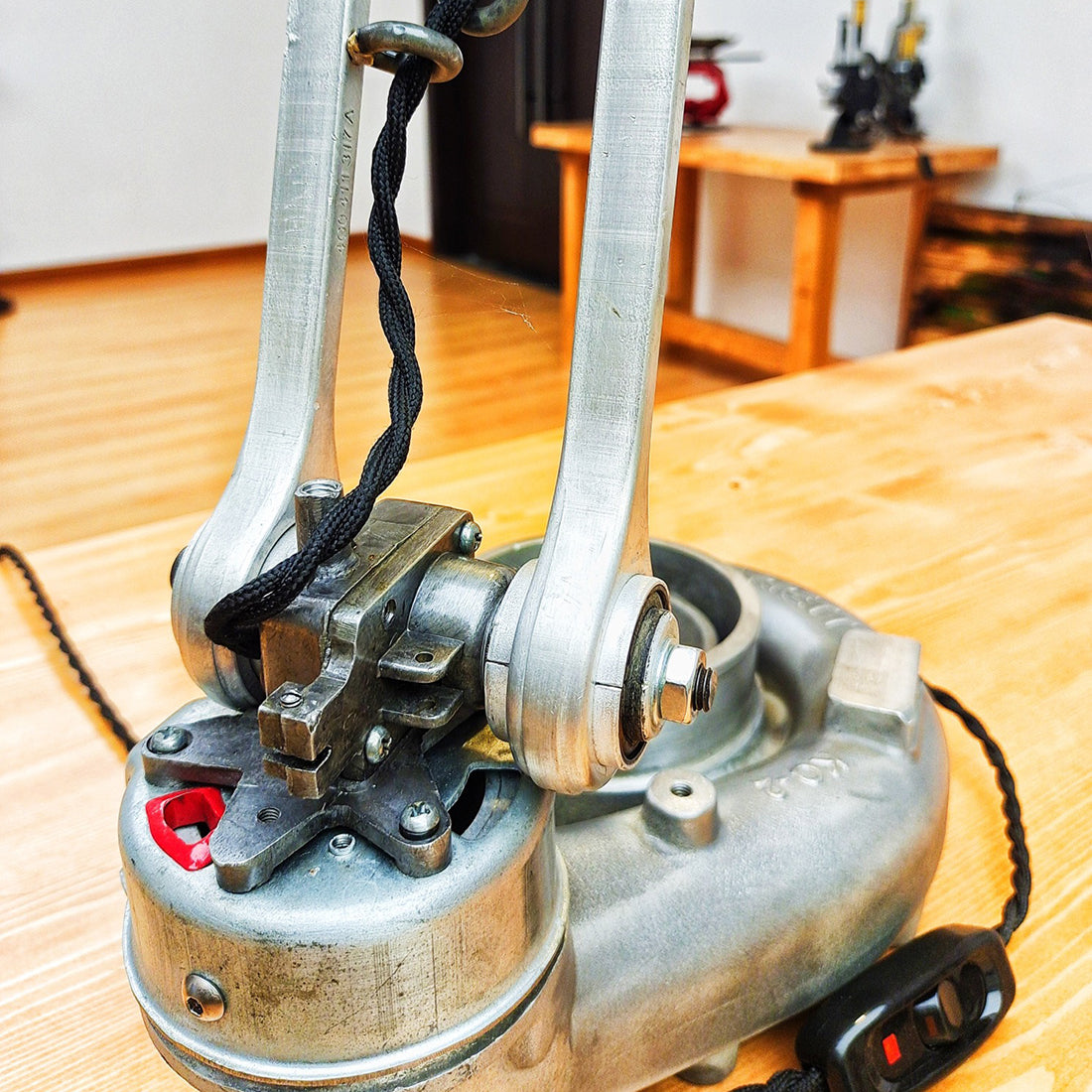This close-up photograph features the bottom part of an old-style, industrial machine, possibly a sander or wood polisher, made primarily of stainless steel or cast aluminum. The central focus is on the round metal base and two vertical handles extending upward. The left handle has a black cable plugged into it, trailing down to the base and attaching to a black metal bracket with a gear mechanism, while the right handle features a rubber gasket at its base and is otherwise plain. A distinctive black on-off switch and twisted black wiring are also visible. The machine sits on a light brown wooden table, suggested to be recently sanded or polished given its refined appearance. In the blurred background, against white walls and a red baseboard, is a polished wooden floor and a light wood credenza with vases and sculptures. A black wooden door is also noticeable amidst the clear and bright setting.